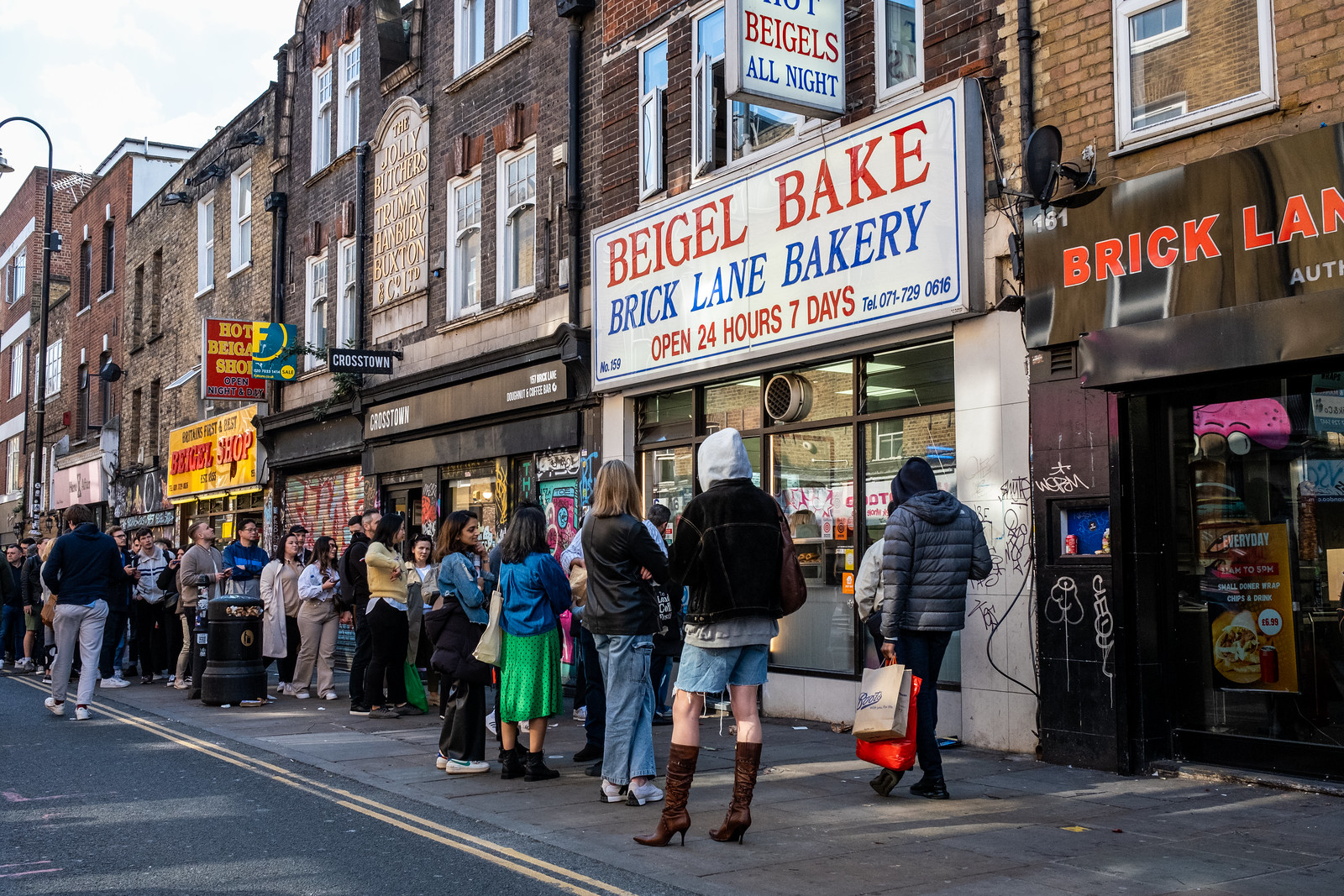In this bustling city street scene, a photographic image captures a long line of at least 30 people stretching down the sidewalk, all eagerly waiting outside the iconic "Beigel Bake, Brick Lane Bakery." The bakery's striking white-brick facade prominently displays a bold sign reading "B E I G E L Bake. Brick Lane Bakery. Open 24 Hours, 7 Days. Telephone 071-729-0616." Above this is another illuminated sign proclaiming "Hot Bagels, All Night," once again using the unique B-E-I-G-E-L spelling. Next door, a storefront with a black-and-red sign reads "B R I C K L A N E," adding to the charm of the area.

Shops like "Crosstown" and "Bagel Shop" line the street at ground level, while the second-floor apartments show an old plaque with the inscription "Jolly Brothers Truman Hanbury Buxton and Company LTD," hinting at the area's history. Despite some graffiti adding to the gritty, urban feel, the area's vibrancy is unmistakable.

Among the people in line, varied fashion choices stand out: a woman in a black jacket, blue jean shorts, and knee-high boots; another person in a gray parka with both a brown shopping bag and a red bag; a woman with folded arms, clad in a black jacket, blue jeans, and gray sneakers; and a person wearing a green skirt, blue jacket, and black shoes. Notably, an Indian woman sports a denim jacket and black shoes, while diverse outfits include yellow-and-black attire, blue-and-khaki combinations, raincoats, and various colored shirts and pants.

The scene is complete with a street light in the background and a sense that this locale is alive and thriving, perhaps reminiscent of New York City or a similar metropolitan area.